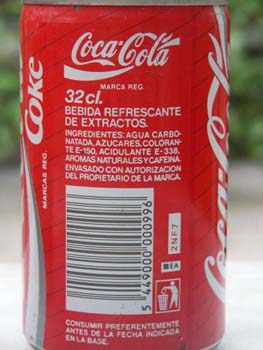This rectangular, portrait-oriented photograph captures a close-up view of the side of a red Coca-Cola can. The iconic white Coca-Cola logo prominently spans the top and the right-hand side of the can. Alongside the logo, text in a foreign language lists the ingredients. The lower portion of the can also features a barcode and a recycling symbol, emphasizing its consumer-friendly design. The can is set against an intriguing two-tone background: the bottom half is light gray, transitioning into a dark green hue in the top half, which adds a striking visual contrast to the image. The photograph meticulously showcases the details and branding of the Coca-Cola can, set in an artistically rendered environment.